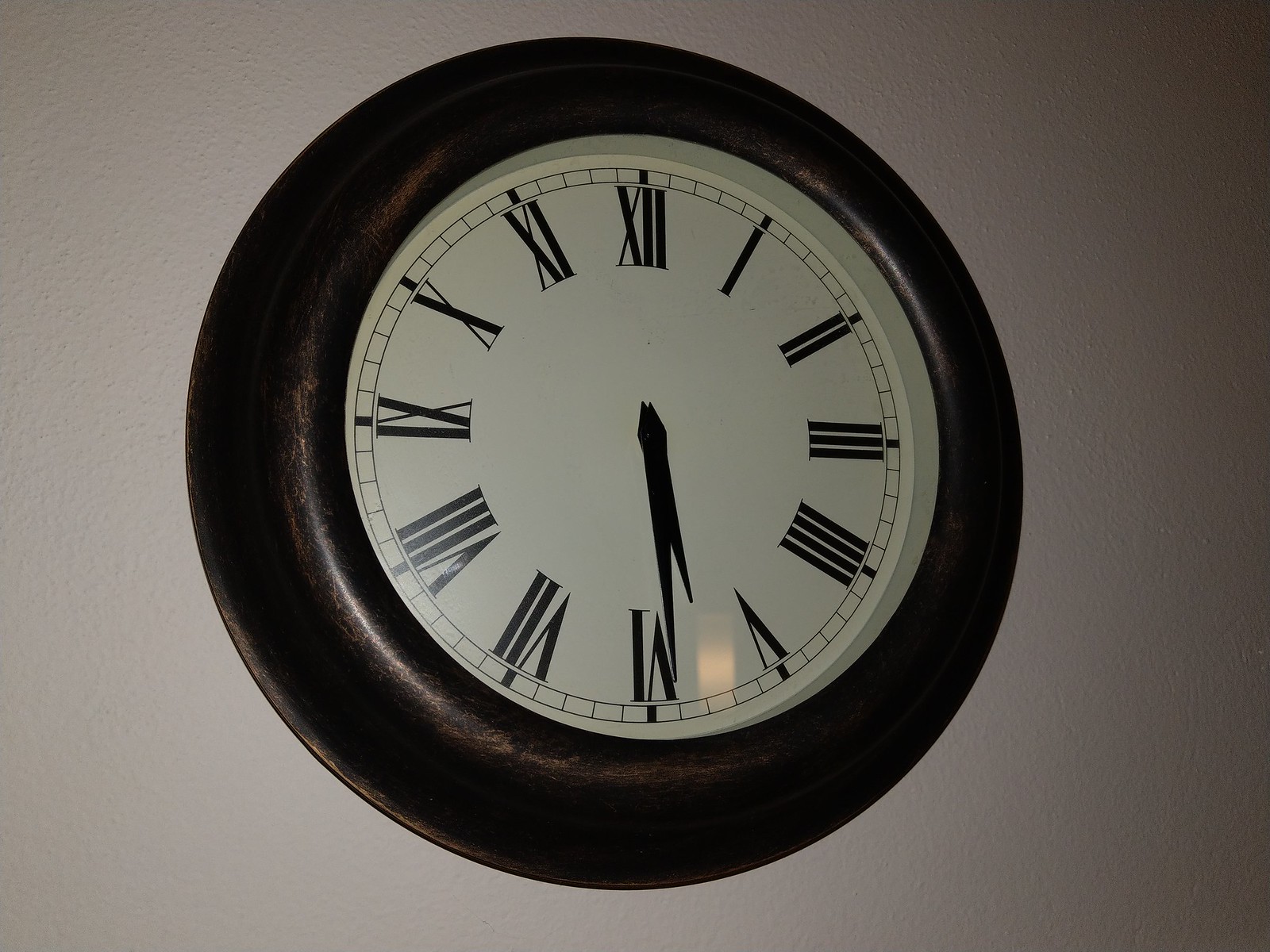This image showcases a simple yet elegant clock mounted on a wall, set against a medium gray background that may be the result of ambient lighting, possibly from a flash or a nearby lamp. The clock features a prominent, thick black frame with a slightly curved design, adding to its classic aesthetic. The face of the clock is a clean, minimalist white, adorned with tall serif Roman numerals to denote each hour. Positioned at the center, the clock hands point downward, indicating the time is approximately 5:30. The overall composition emphasizes the clock's timeless elegance and understated sophistication.